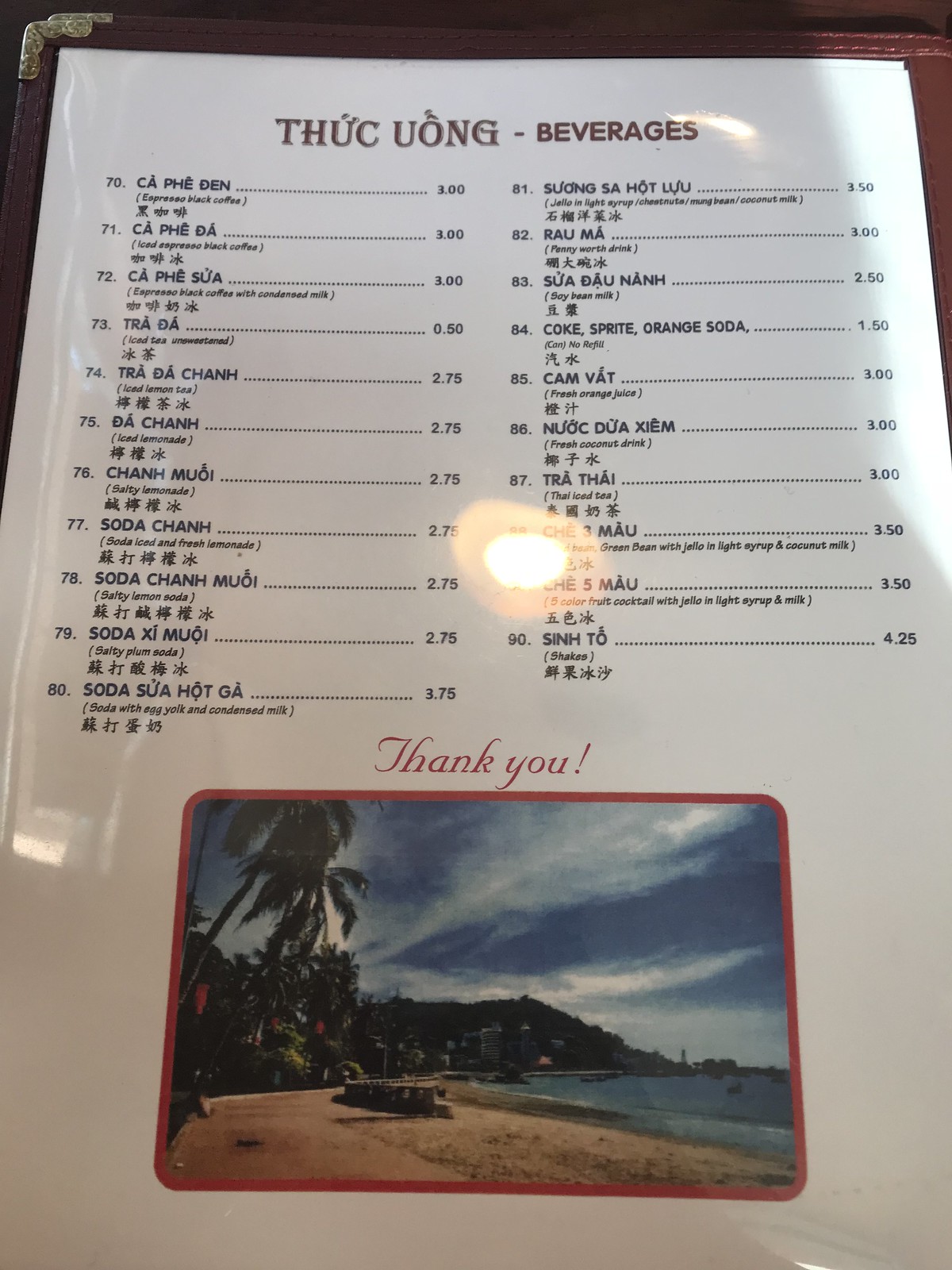In this picture, a white menu is displayed within a possibly dark reddish brown or burgundy case, which features intricate gold detailing in at least one corner. The menu itself is placed on a dark wooden surface, either a table or a counter, which adds a contrasting background. At the very bottom of the menu, there is an image depicting a beach scene with water, buildings in the distance, a sky filled with clouds, and palm trees, infusing a touch of tropical atmosphere. 

The header of the menu is written in an Asian language, possibly transliterated as "thong th-uc" and "u-o-ng," followed by "beverages." The menu is segmented into two sections, with items numbered 70 to 80 on the left and 81 to 90 on the right. Although some beverage names are recognizable, such as various sodas, many are in a language that is difficult to identify. The prices, ranging from $2.50 to $4.25, are quite reasonable.